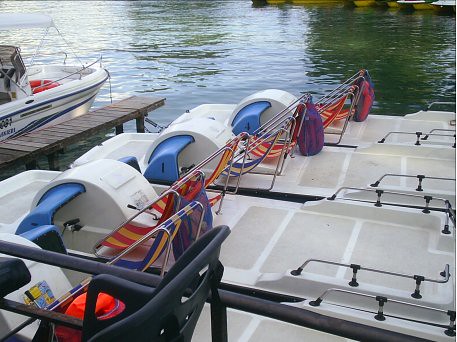The image depicts a scene at a lake dock featuring a row of paddle boats, parked nose-first against a long, brown wooden dock. In the foreground, there are four paddle boats, three of which are fully visible while one is partially obscured. Each boat is equipped with mesh net seats, fashioned in red and yellow striped fabric for one pair and blue and yellow striped fabric for another. These seats recline and face partially forward towards a blue protective cover that houses pedals beneath it. Between the two seats, there's a raised white plastic section, and behind them lies an empty white plastic deck. At the back of the boats, there are visible gray handlebars. The greenish-blue water of the lake stretches out in the background, next to a separate white and blue motorboat docked alongside. These paddle boats are clearly rented for leisure, allowing people to pedal out into the lake for relaxation or as a platform to swim from.